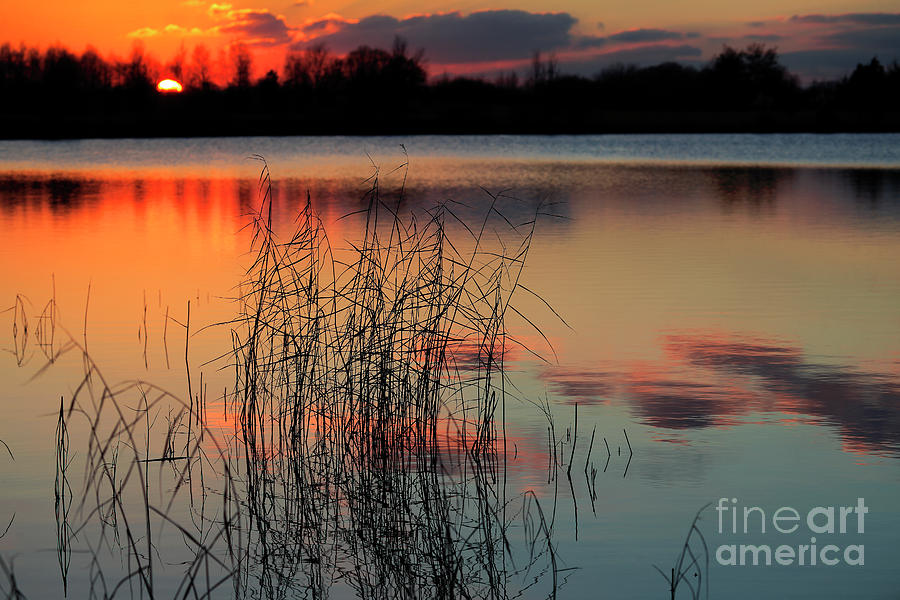This photograph captures a breathtaking sunset over a serene lake, with rays of the setting sun illuminating the scene. Near the horizon, a glowing orange sun descends behind a silhouetted tree line. The sky presents a majestic gradient, transitioning from deep red at the horizon to vibrant orange, yellow, and subtle hints of purple and blue higher up, with wispy clouds stretched across the expanse. The tranquil lake mirrors the sky's rich hues, blending orange, yellow, and ripples that shift to silver, blue, and white closer to the foreground. Along the water's edge, some tall wild weeds grow, adding an element of natural beauty. The composition is signed with a watermark reading "Fine Art America" in the bottom right corner.